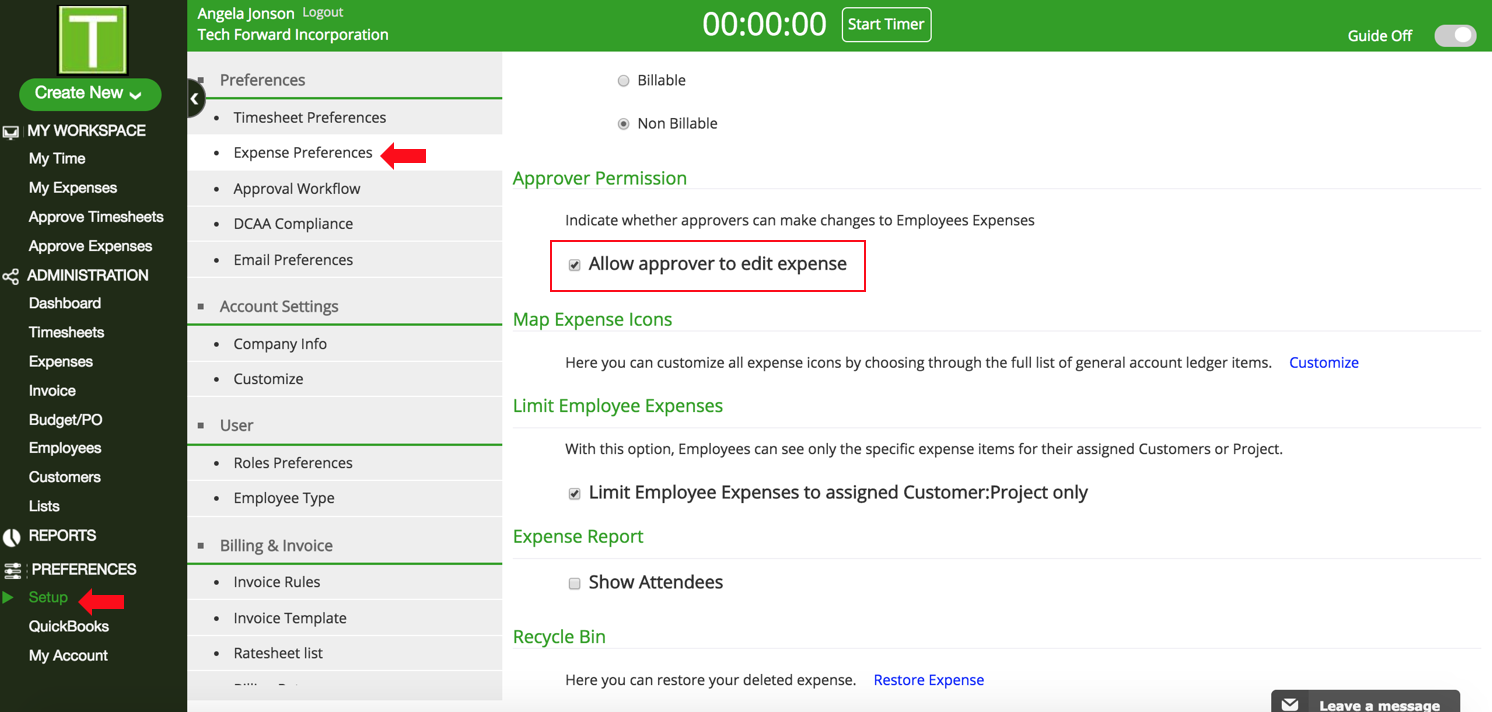The website interface depicted in the image appears to be an administrative dashboard for workplace management, featuring a simple and utilitarian design. On the left side of the screen, there is a prominently displayed dark green column with various navigational options. At the top of this column is a large white "T" inside a green box, followed by a green button labeled "Create New" in white text.

The navigation bar includes sections for "My Time," "My Expenses," "Approved Timesheets," and "Approved Expenses," suggesting functionalities related to time and expense management. Additionally, there is an "Administration" section with further subsections such as "Dashboard," "Timesheets," "Expenses," "Invoices," "Budgets," "Employees," "Customer List," and "Reports," all of which are capitalized for emphasis. The "Preferences" section is also capitalized and situated just below the reports. Additionally, there is a "Setup" area indicated by a right-pointing arrow, leading to options like "QuickBooks," which suggests some integration capabilities.

In the top right corner of the dashboard, the current user "Angela Johnson" is logged in, with an option to log out. Angela Johnson's workplace information, "Techfort Incorporation," is displayed beneath her name, alongside her designation. The interface shows various user preference settings, including "Timesheet Preferences," "Expense Preferences," "Account Settings," "Users," and "Billing & Invoices," with some options featuring arrows for further sub-options.

There is also a green top bar displaying "Techfort Incorporation," with additional tools like a timer, billable/non-billable toggles, and approval permissions. This section includes options such as "Approval Permission" which allows approvers to edit expenses, indicated by a checkmark inside a red box. Other settings like "Map Expense Icons," "Limit Employee Expenses," "Expense Report," and "Show Attendees" are present, each with corresponding checkboxes, with some options enabled and others disabled.

At the bottom right corner of the screen, there is a "Leave a Message" button for user support or feedback.

Overall, the image portrays a detailed, comprehensive administrative dashboard tailored for workplace management, particularly focusing on time and expense tracking functionalities.